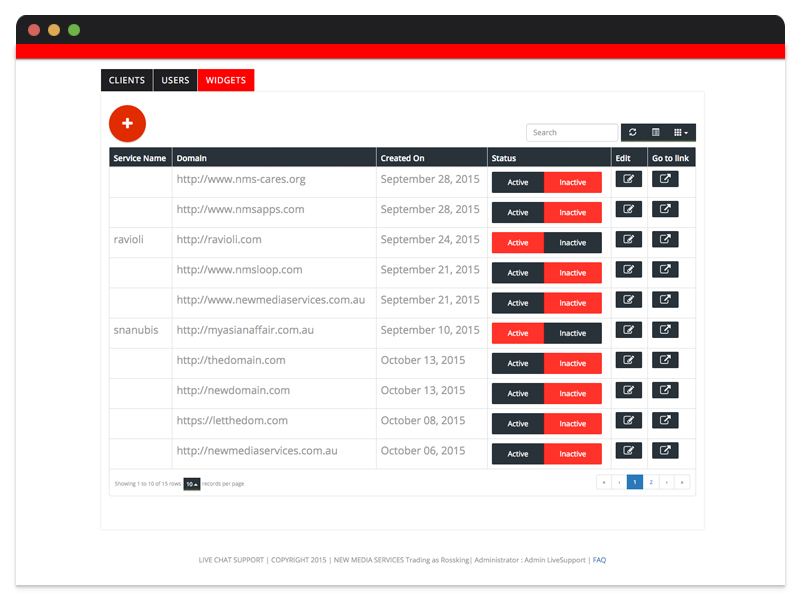The image depicts a webpage interface with a detailed layout. At the top, there is a horizontal black bar featuring three colored dots—red, orange, and green—aligned from left to right. Below this black bar is a bold red stripe running across the page.

The primary navigation area highlights categories labeled "Clients" and "Users," enclosed in a black box. The "Widgets" option appears to be selected, indicating the current view. 

Central to the page is a prominent red circle containing a white plus sign. The interface is divided into columns, each labeled as follows: Service Name, Domain, Date Created, Status, Edit, and Go To Link. Within the 'Edit' column, a blue box is highlighted.

At the bottom of the page, there is a footer section displaying "Live Chat Support," copyright information labeled as "Copyright 2015," and "New Media Services," noted as "Trading as Rosking Administrator." Additionally, the footer includes "Administrator Live Support" and a reference to "Fax."